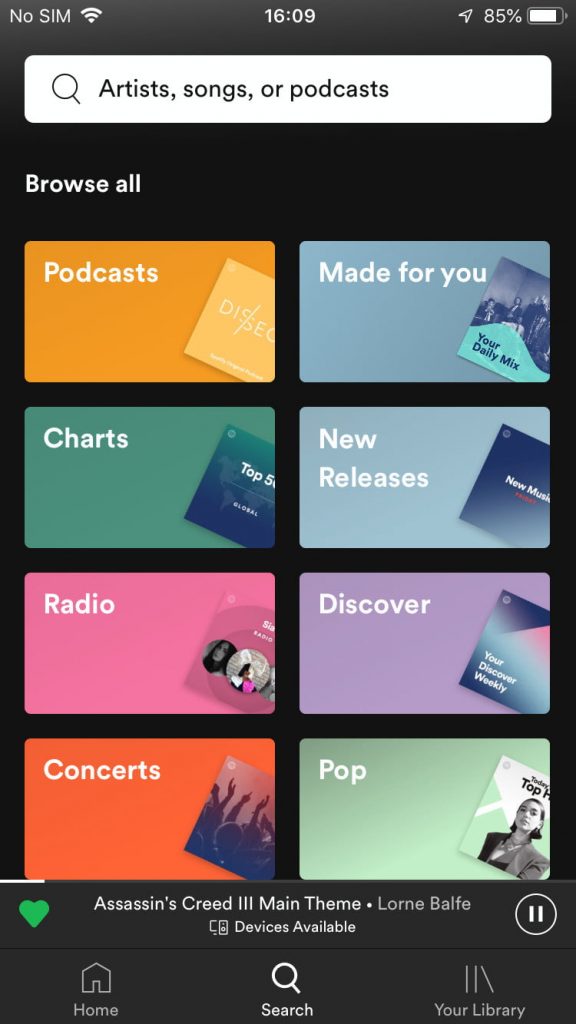This is a detailed screenshot from the Spotify app interface on a mobile device. 

In the top left corner, there is an indicator that reads "No Sim" accompanied by a cellular signal icon. The time displayed at the center of the top bar is 16:09, and on the far right, the battery level is shown to be at 85%.

Below the top bar, there is a white rectangular search bar with a magnifying glass icon, featuring the text "Artist, Songs, or Products."

Underneath the search bar, there is a "Browse All" section set against a black background. This section is divided into two columns filled with eight different music categories:

- **First Column:**
  1. **Podcasts:** Orange background.
  2. **Charts:** Green background.
  3. **Radio:** Pink background.
  4. **Concerts:** Red background.

- **Second Column:**
  1. **Made For You:** Light blue background.
  2. **New Releases:** Lighter blue background.
  3. **Discover:** Purple background.
  4. **Pop:** Lime green background.

Currently, the song "Assassin’s Creed II Main Theme" by Lauren Belf is playing. Next to the song title, there is a green heart icon, indicating it is liked, and a pause button.

At the bottom of the screen, there are three icons for navigation, including a "Home" icon, a "Search" icon, and a "Your Library" icon.